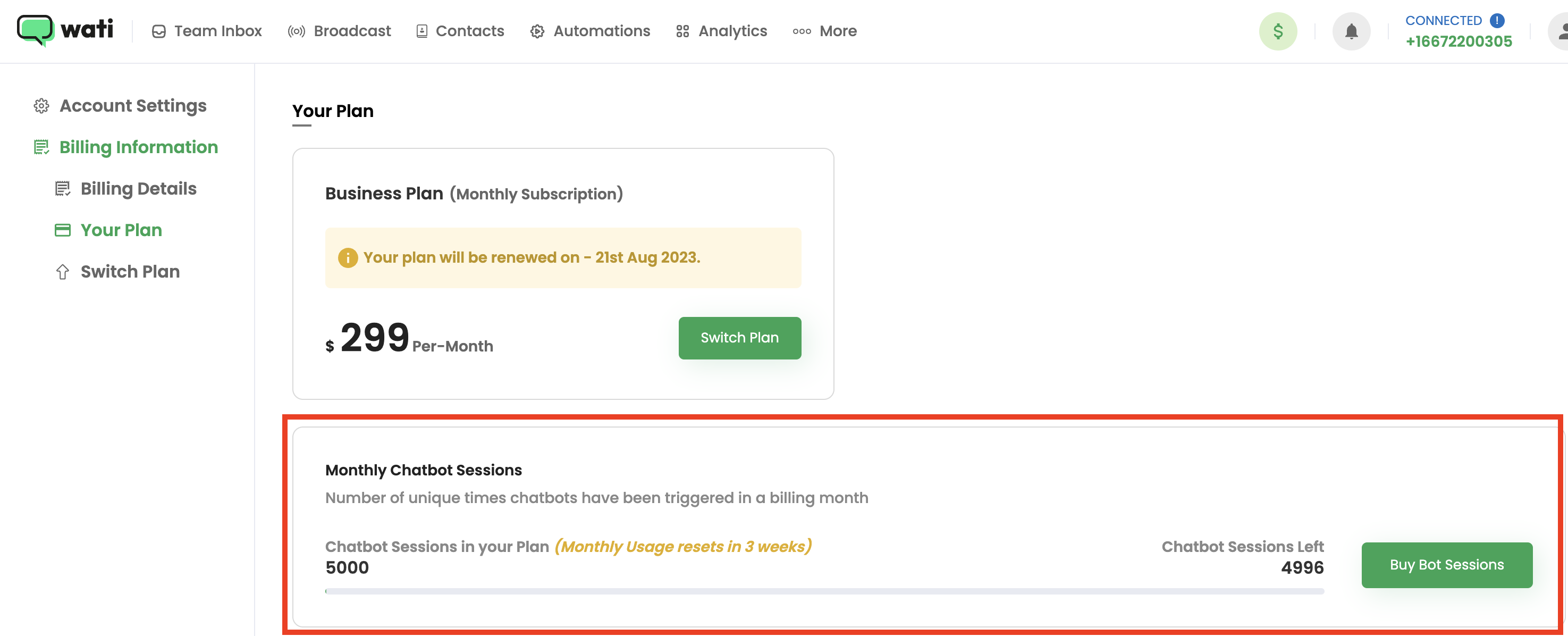The image displays the billing details for a "Business Plan" subscription, which costs $299 per month. Key information includes the option to switch plans and the renewal date, set for August 21, 2023. It also highlights the number of chatbot sessions available under the current plan, specifying how many unique times chatbots have been activated during the billing period. The monthly usage statistics show that the usage will reset in three weeks, and there are 4,996 chatbot sessions remaining. Additionally, there is an option to purchase more bot sessions if needed.